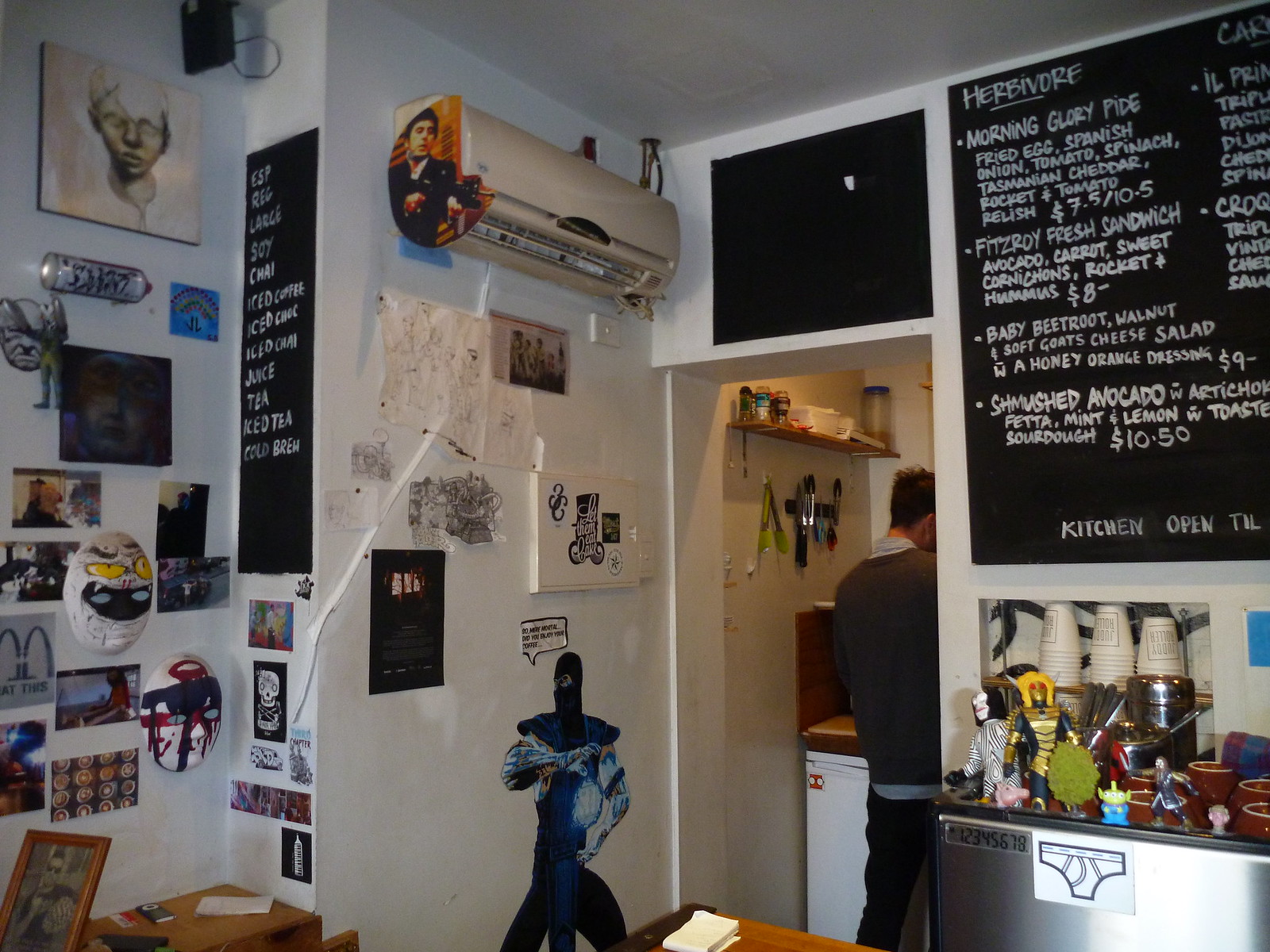The photograph, taken indoors in a rectangular format just slightly wider than tall, captures an eclectic scene in what appears to be a quirky restaurant or café. The walls, painted a pristine, snow-white reminiscent of a porcelain finish, serve as a stark backdrop to the crowded array of posters, signs, paintings, and pictures that saturate the space, creating a vibrant collage of art and knickknacks.

To the right of the image, a partial view of a man with light skin and short brown hair is visible as he stands with his back to the camera. He wears a combination of garments—a gray long-sleeve shirt or sweater over a blue shirt, paired with black jeans. Positioned near a door in a nook-like area, he seems engaged in preparing a drink or attending to something on a shelf that houses tongs, spices, and other items.

Adjacent to the man, a black chalkboard menu occupies a section of the wall, displaying various offerings in white print, including "Herbivore Morning Glory Pie," "Fitzroy Fresh Sandwich," "Baby Beetroot Walnut and Soft Goat's Cheese Salad," and "Smushed Avocado with Artichoke," with additional ingredients and prices noted beneath each entry. Beneath the chalkboard, a silver mini-fridge adorned with a quirky sticker resembling white underwear stands next to a countertop cluttered with cups, action figures, and assorted objects.

On the left side of the room, more peculiar decorations come into view—a collection of masks, pictures, and standout characters such as an image of Al Pacino and figures from video games, contributing to the room's distinctive, eclectic ambiance.